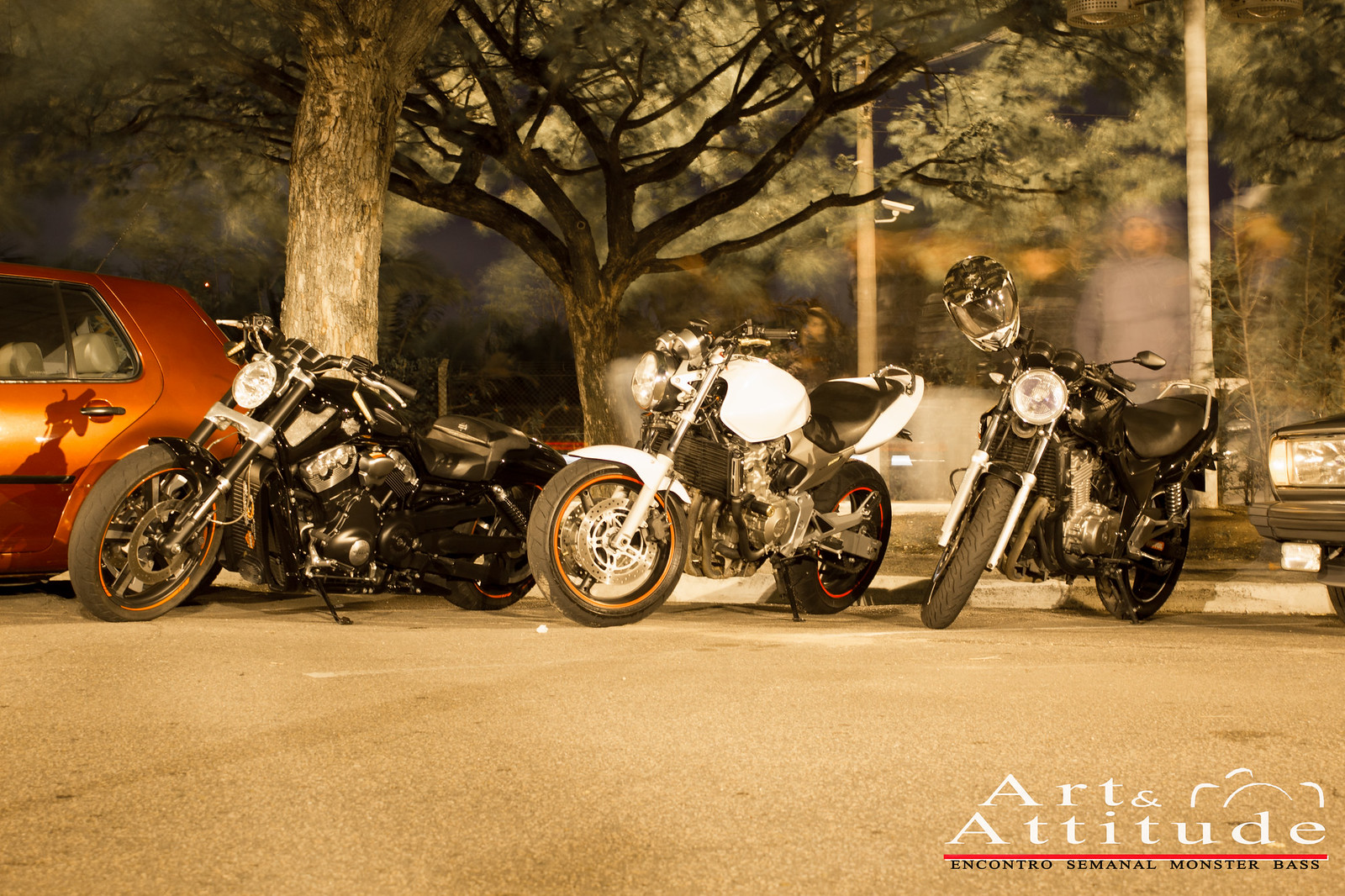This image depicts three motorcycles parked side-by-side on a gravel street, positioned next to an orange car on the left. Each motorcycle is angled slightly differently, with a black motorcycle closest to the car, followed by a more silver-colored motorcycle, and then another black motorcycle on the far right. Partially visible on the right side of the image is the headlight of a black car. Beneath the motorcycles, white letters spell out "Art and Attitude" followed by an orange line and black letters reading "Encontro Seminole Monster Bass." The scene has a brownish tint and appears to be taken either at dusk or dawn, with light coming from an ambiguous source. In the background, trees with leaves are visible, and there is an indistinct, ghostly presence of a man in a gray hoodie and possibly a woman with long hair. Additionally, the far-right motorcycle has a blurred figure, suggesting a person with discernible facial features.